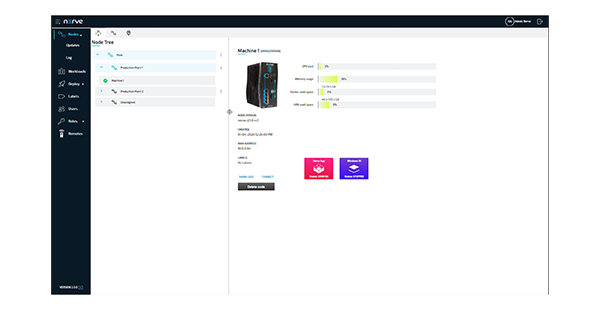Displayed in the image is a vertically oriented PC tower featuring distinct design elements. The left side of the tower diverges from the usual straight edge, presenting a unique curved silhouette. The front panel of the tower is primarily gray, adorned with a combination of blue and black buttons that provide contrast. The curved portion of the tower is black, adding to the aesthetic appeal.

To the far left of the image, there is a vertical black column containing various filter options. Adjacent to this, slightly to the right, there appears to be a node tree or a similar interface with five selectable options. The top two of these options are highlighted in light blue, while the remaining three are in gray.

Positioned next to the PC tower itself is a section with four indistinct bars, accompanied by some textual identifiers that are not entirely legible. This combination of elements suggests a detailed interface, possibly for managing or monitoring the PC tower or a related system.